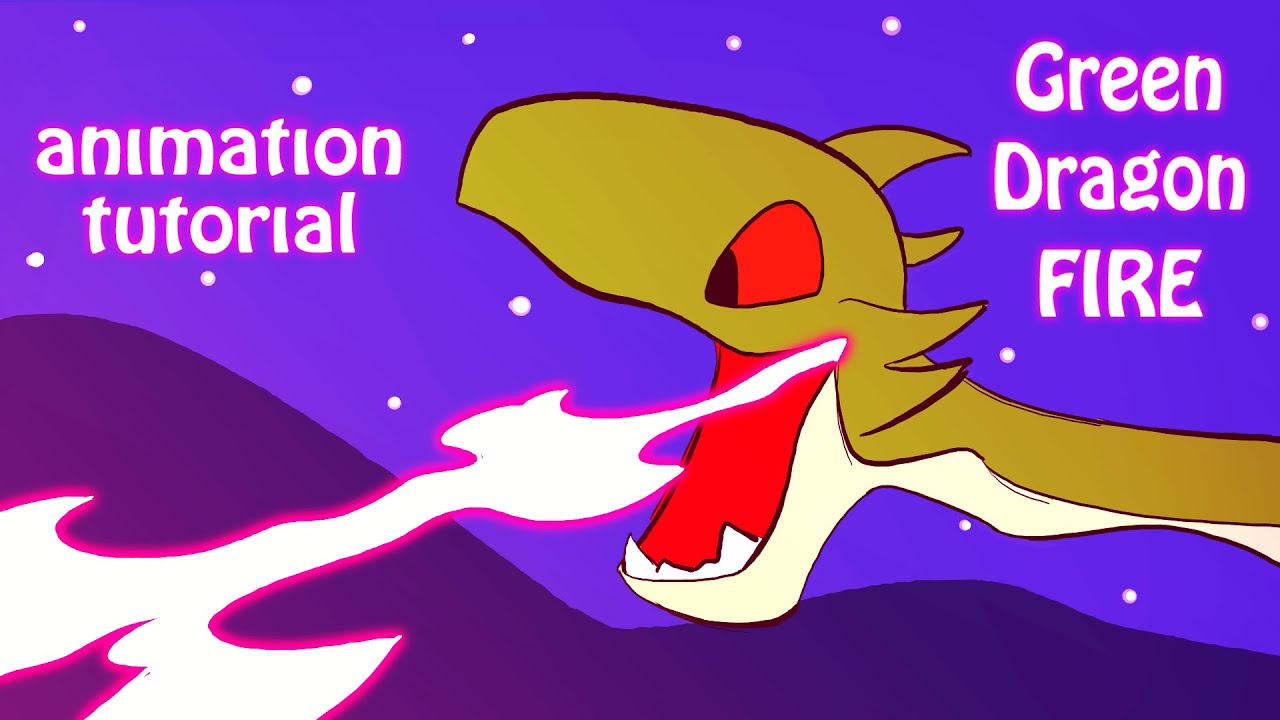This cover graphic for an animation tutorial, titled "Green Dragon Fire," features a detailed illustration of an olive or forest green dragon with a lighter, off-white underbody. The dragon has red eyes with black pupils and a red interior to its open mouth, from which it breathes out glowing white and pinkish-red fire. The background is a two-tone blue and purple gradient, mimicking a night sky with white dots resembling either stars or snow. The upper part of the background is lighter with white circles, while the bottom transitions to a darker, purplish-blue that suggests a silhouette of hills or mountains. At the top of the image, glowing white text bordered in purple reads "Animation Tutorial" and "Green Dragon Fire."